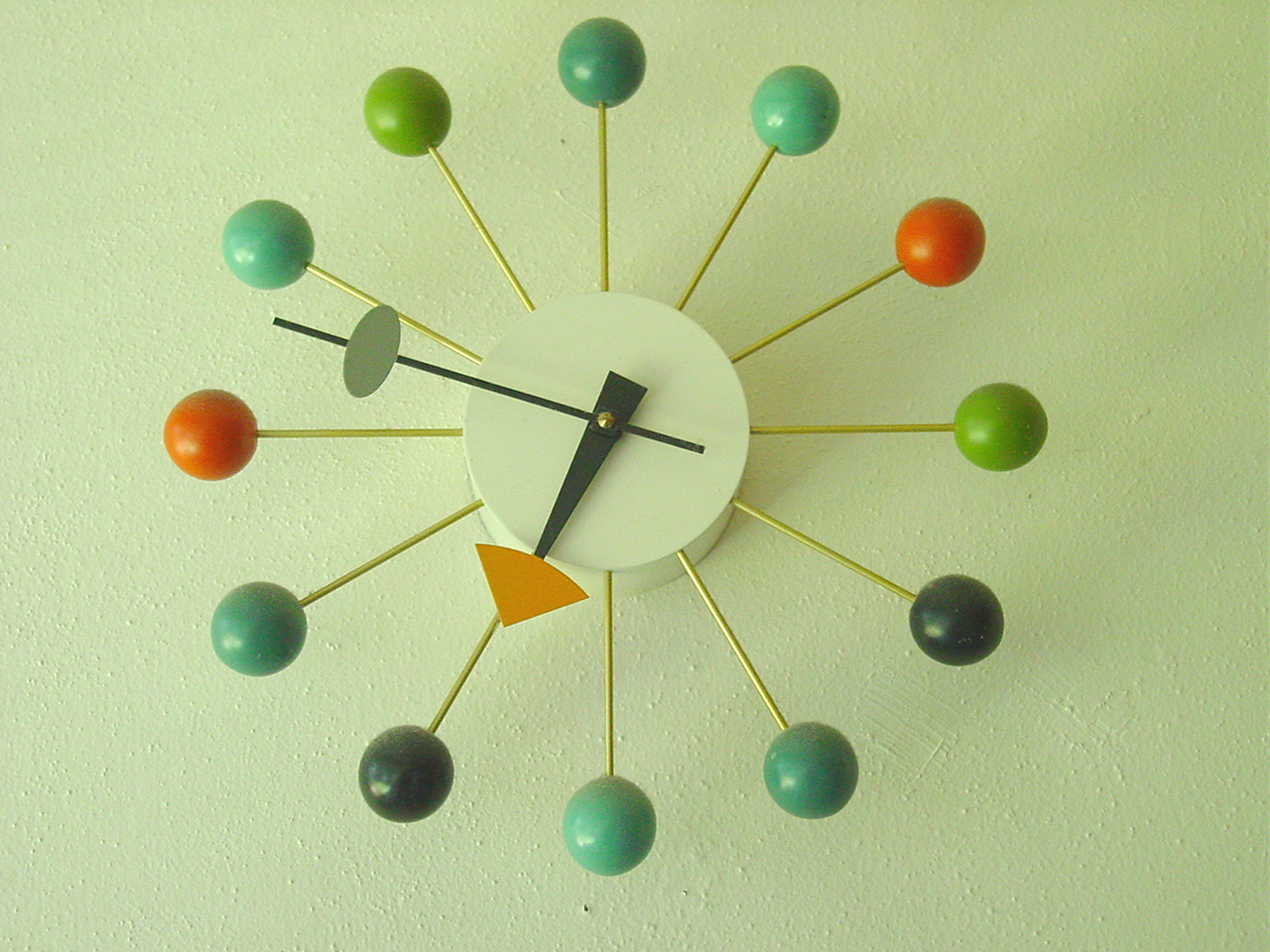This image showcases a striking mid-century style wall clock set against a pale green wall. The clock features a round white base, reminiscent of a hockey puck, housing two distinct hands: an hour hand with a mustard yellow triangle pointer and a minute hand with a gray oblong pointer. Extending from the base are twelve gold sticks, each crowned with a marble-like ball in place of traditional numbers. These balls vary in colors, including different shades of green, black, and two shades of orange, resembling lollipops or cake pops. The unique and colorful design elements combine to create a modern, yet nostalgic timepiece.